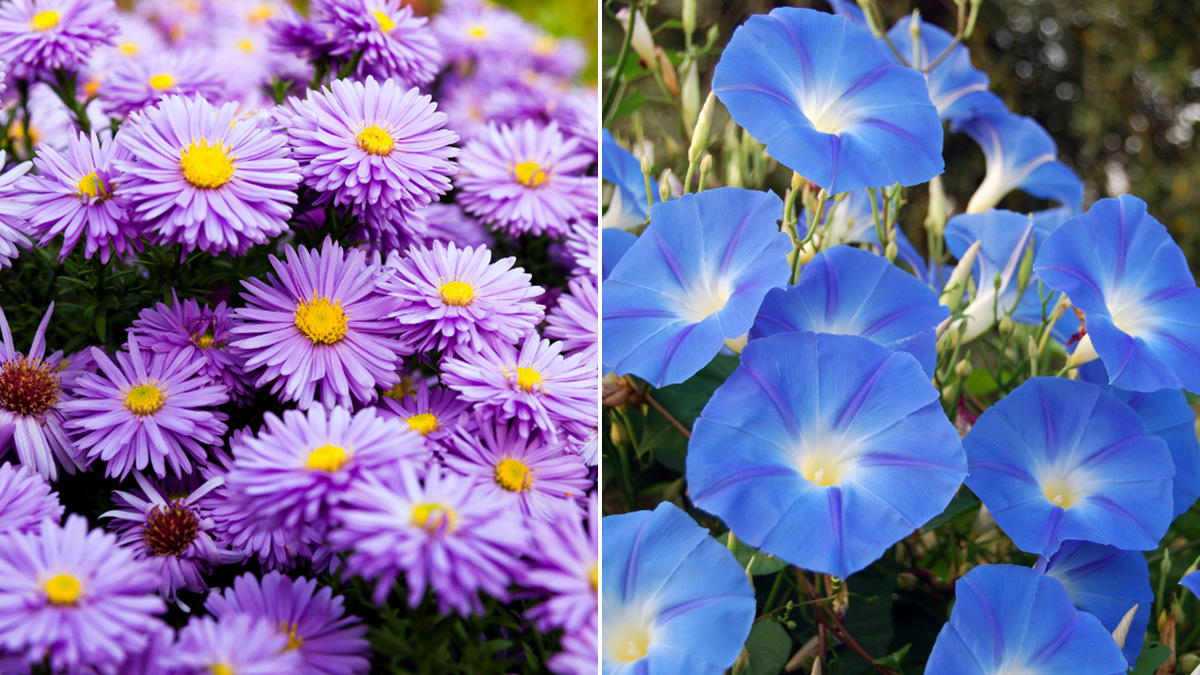This image features two side-by-side close-up photographs of different flowers, each taking up half of the frame. On the left, there are purple flowers with thin, delicate petals radiating from a yellow center, resembling dandelions with purple petals. Some flowers also have a darker reddish hue in the middle. The blossoms are well-focused in the center of the image, with a slightly blurred upper portion and visible green stems and a hint of grass in the background.

On the right, the photograph captures blue flowers with a unique structure; the petals form an umbrella-like shape with no distinct separations, featuring a deep yellow center that transitions to white before blending into a vibrant blue. The petals exhibit subtle purple indentations along their curved edges. These flowers are more densely clustered toward the bottom of the image, where the focus is sharp, with the upper right corner appearing slightly blurry. Green stems and leaves are faintly visible in the background of both photos, grounding the natural composition.